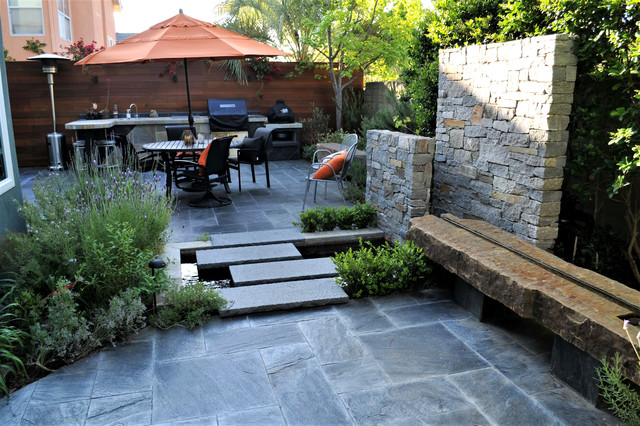This color photograph captures an elaborate backyard patio setup with multiple levels and detailed landscaping. In the foreground, there is a stone patio section made of grey slate, featuring a small water feature that can be crossed using four rectangular stone slabs. On the right side of the pathway, there are two freestanding walls made of a combination of grey and rust-colored stones, along with a stone bench also made of rust-colored stone. Adjacent to these structures is a small garden area with lush green shrubs and purple flowers.

Behind this, a second stone patio area extends into the background. It showcases a circular table surrounded by chairs and topped with an orange umbrella. Nearby, there's an outdoor grill station equipped with a granite countertop and an additional sink with a faucet. A large stainless steel light fixture is mounted to the left, illuminating the space.

A brown wooden fence forms the backdrop of this well-designed patio, with a pink house visible beyond it, indicating an urban environment. The ambiance is further enriched by various outdoor amenities, making it a versatile and inviting outdoor setting.